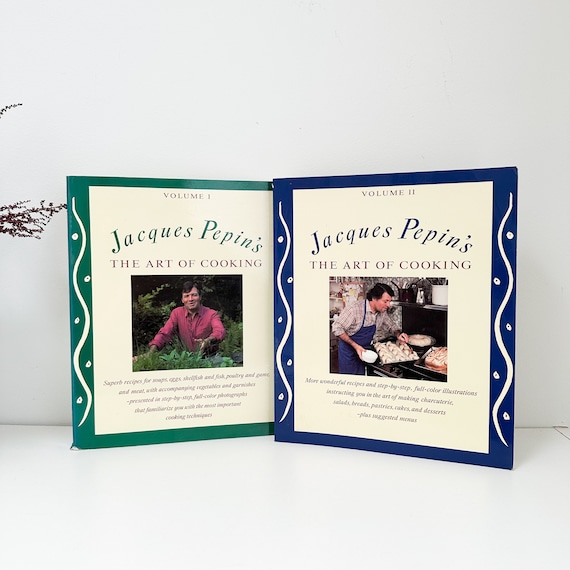This image features two covers of Jacques Pépin's "The Art of Cooking." On the left, Volume 1 displays a picture of Jacques Pépin in a light pink shirt with a green border around the cover. He is depicted outdoors, standing over lush bushes, with his hand poised as if to gather herbs or vegetables. Below the photograph, a story is present, though the text is too small to discern. On the right, Volume 2 is bordered in blue and shows Pépin indoors, in a kitchen setting. He is wearing a long-sleeved collared shirt with the sleeves rolled up, and a blue cooking apron. Pépin is holding a circular white bowl and tending to several dishes, seemingly placing or removing them from the oven. Both volumes prominently bear the title "Jacques Pépin's The Art of Cooking" at the top, with additional small text under each photo.